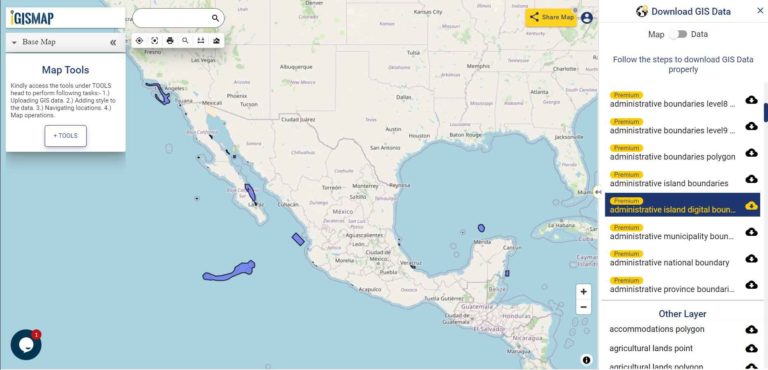The image depicts an interactive Geographic Information System (GIS) map, prominently labeled "GIS Map" in blue at the upper left corner. Beneath this title is a "Base Map" label, followed by a "Map Tools" section. Instructions in this section prompt users to "kindly access the tools under Tools" to perform tasks such as uploading GIS data, adding styles to the data, and navigating locations for map operations. A "Plus Tools" button is also present for additional functionalities.

The map displayed covers the lower half of the United States, extending from Illinois in the north to Mexico in the south. It includes parts of Central America like Honduras and surrounding islands. Not all states are visible, but key areas such as Texas and Mexico are prominent. 

On the right side of the map, there is a "Download GIS Data" section that offers various data sets available for download. Additionally, an "Other Layers" section is present, presumably for layering different GIS data types over the base map. 

This GIS map interface allows users to input locations and download specific map data tailored to their needs, with the current view primarily highlighting the geographic regions of the United States and Mexico.